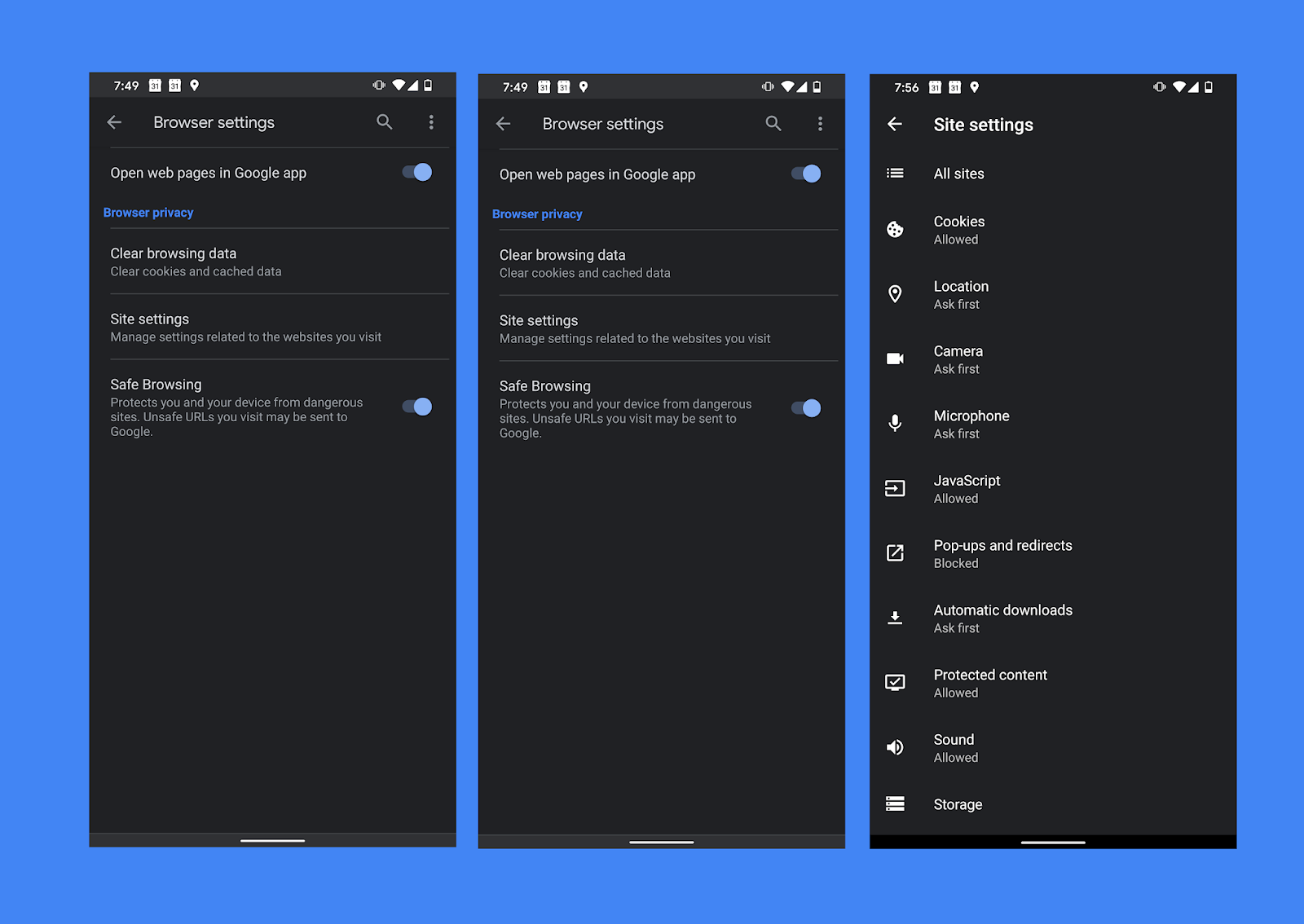The image displays a large blue background with three black smartphone screens aligned vertically. 

**First Screen:** The first screen shows a browser settings interface. At the top, there is a left arrow, a magnifying glass icon, and a three-dot menu icon. Below this, several options are listed: "Open with pages in Google app," "Browser privacy," "Clear browsing data," "Site settings," and "Safe browsing." A small blue dot appears to the right, indicating a toggle option.

**Second Screen:** The second screen mimics the first with slight variations. It again features the browser settings at the top, including "Open web pages in Google app." Below are similar options: "Browser privacy," "Clear browsing data," "Data settings," and "Safe browsing," each accompanied by a blue sliding toggle button.

**Third Screen:** The third screen focuses on "Site settings," indicated by a left arrow. It lists various options: "All sites," "Cookies," "Location," "Camera," "Microphone," "JavaScript," "Pop-ups and redirects," "Automatic downloads," "Protected content," "Stand and storage." Each screen ends with a white line at the bottom.

This detailed view showcases the intricate settings available within a browser's interface on a smartphone.